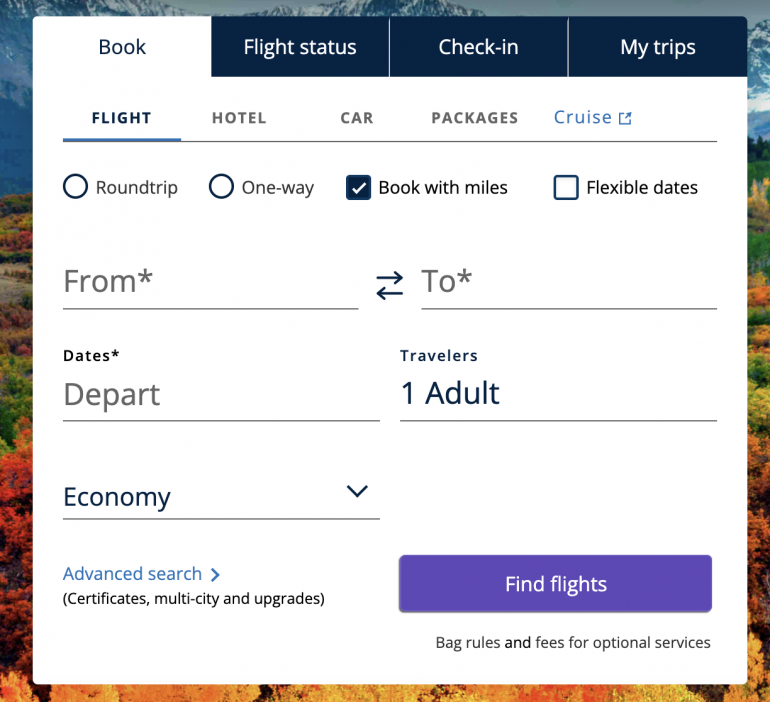The image depicts a web page where a user is in the process of booking a flight. The interface features a clearly organized layout with various options and fields to facilitate the booking.

At the top, a tab labeled "Book" is highlighted in white, indicating the current section the user is in. Below this, there's a menu with several options. The "FLIGHT" option is prominently displayed in bold, capital letters, underlined, and colored in dark purple to show that it is selected. Adjacent to this selection, other options are listed in gray: "Hotel," "Car," and "Packages." Additionally, a blue option labeled "Cruise" with a share symbol appears on the far right.

A light gray border frames the main booking section, with a dark blue vertical line on the left side. Here, two circular tick boxes are situated: one for "Round Trip" and another for "One-Way." Below these, two square tick boxes are presented. The "Book with Miles" option is selected, marked by a dark blue fill and a white check mark, while the "Flexible Dates" option remains unchecked.

The booking form itself is highly detailed. It includes fields for "From" and "To," both marked with asterisks, indicating they are mandatory. Between these fields, there is a right-pointing arrow, with a left-pointing arrow underneath it. The "Dates" field, also marked with an asterisk and in black font, includes a section for "Depart" written in basic gray sans serif font. Another field labeled "Travelers" shows "1 Adult." Below this, an "Economy" option has a downward arrow, indicating the presence of a dropdown menu for class selection. 

Towards the bottom of the form, a "Advanced Search" link in blue, accompanied by a right-pointing arrow, leads to expanded search options. Under this link, in black text within parentheses, are additional features: "certificates, multi-city, and upgrades."

A large purple rectangular button at the bottom, with white text, invites the user to "Find Flights."